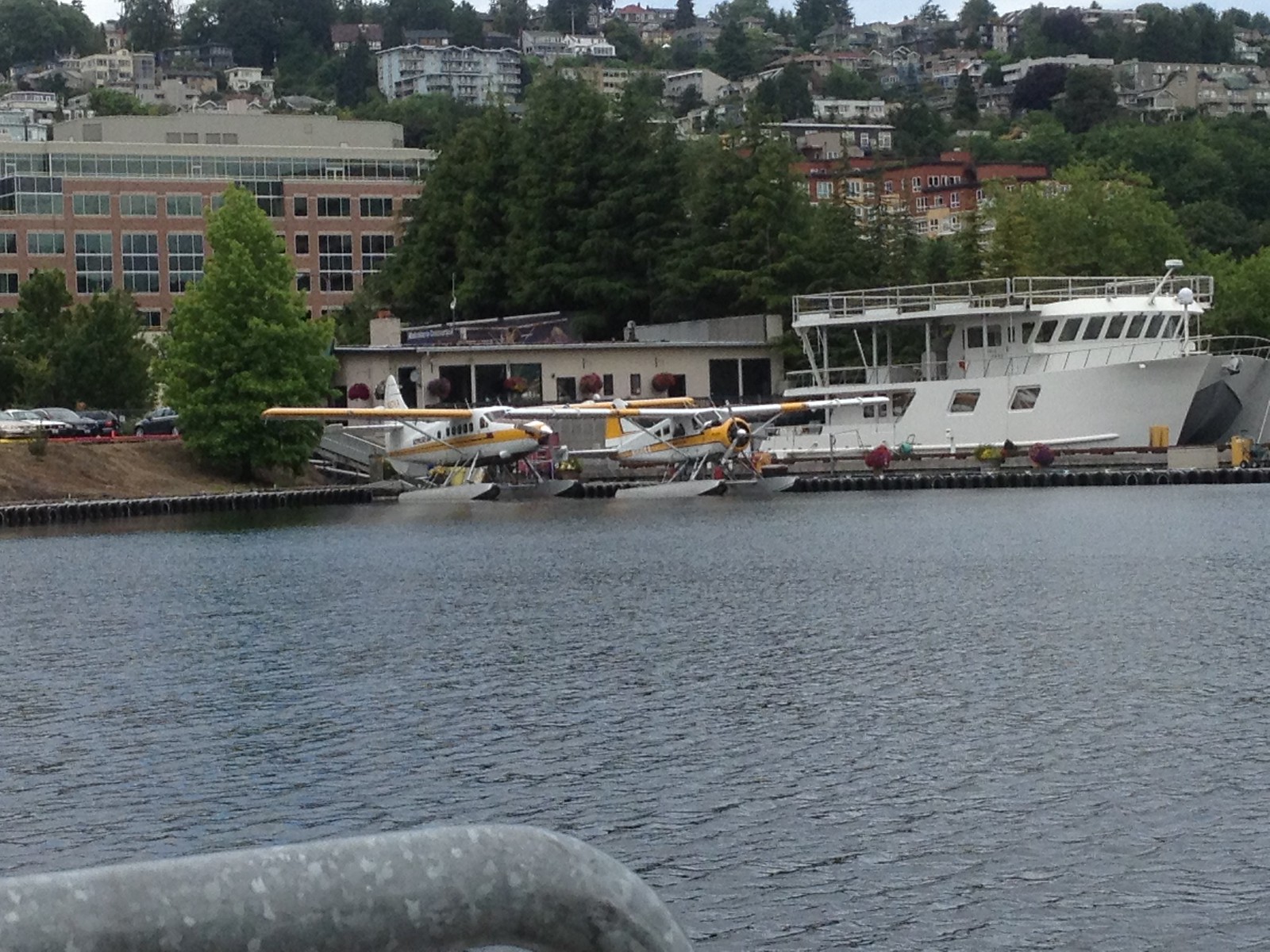The image captures a bustling marina scene, featuring an expansive body of calm, dark water. Dominating the foreground are two yellow and white propeller seaplanes docked closely together. Adjacent to the seaplanes is a large, white, flat-top boat with numerous windows, likely a sightseeing or party vessel. The dock area includes a flat building with large windows, probably serving as the office for the seaplanes. The scenic backdrop features a variety of large trees with light and dark green leaves, leading up to a hillside teeming with buildings in tans, browns, and grays. These buildings rise up the hill, suggesting a town that overlooks the marina. Scattered across the scene are various objects, including a parking lot with cars and a grey metal bar at the bottom edge of the image, indicating the viewer’s position on the opposite side of the water. A sliver of blue sky peeks across the top, completing the vibrant landscape.